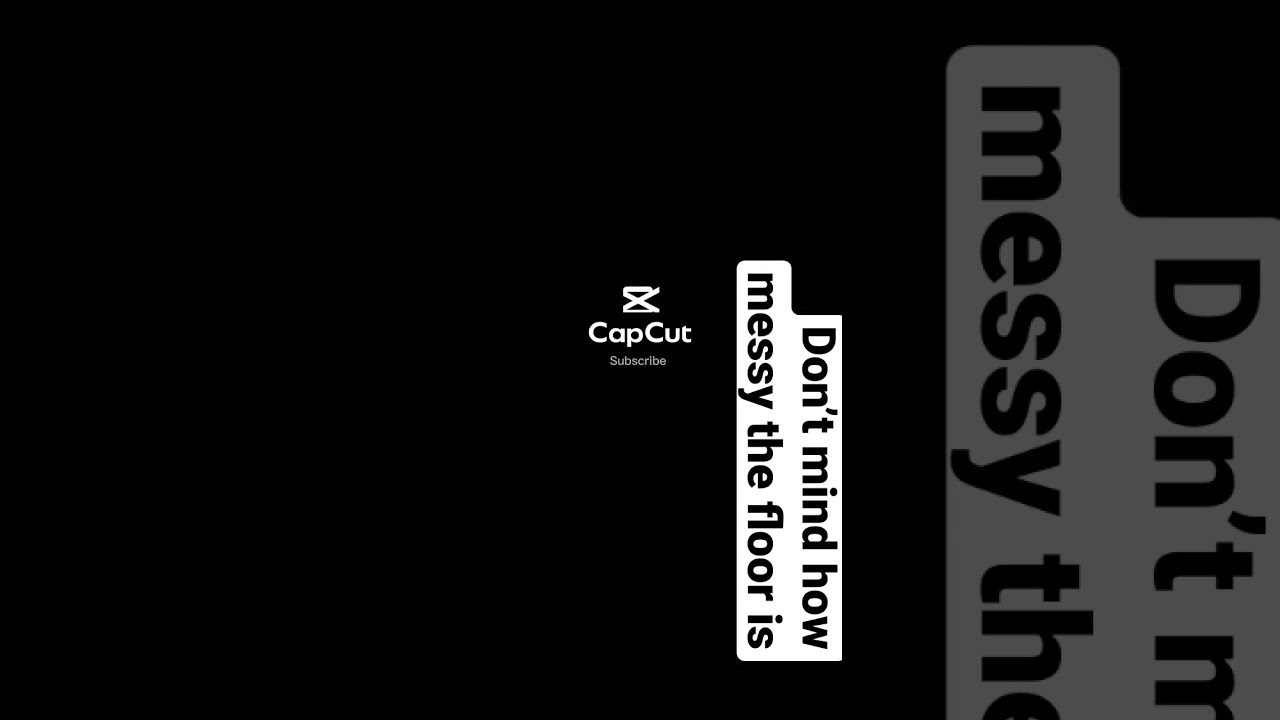The image predominantly features a pure black background. Positioned in the center is a branding section with the text "CAPCUT" in white letters, where both C's are capitalized. Above this, there is a brand symbol consisting of a white X flanked by two horizontal bars. The upper right arm of the X slightly extends beyond the top border. Directly beneath this symbol is a smaller text that says "subscribe."

Towards the right of this central section, there are two white strips of text rotated 90 degrees to the right, making them appear sideways. The top strip, which is shorter, reads in black letters, "don't mind how messy the floor is." This is reiterated by a much larger and partially visible version of the same text, which fades out and extends beyond the bottom right-hand corner of the image. Both text elements align vertically along the right-hand side, creating a layered effect. The image is cleanly sectioned into mostly black areas with these distinct white text and symbol details.